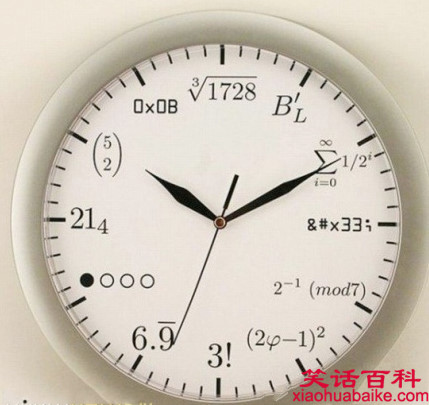Here is a detailed and refined caption for the image:

"This unique clock features a dial divided into 12 primary segments, with smaller divisions in between. Instead of traditional numbers, the face is adorned with various mathematical symbols, European numerals, and capital letters. Adding to its eclectic design, the bottom right-hand corner of the image showcases bright red Asian or Chinese characters alongside an unpronounceable name followed by '.com,' suggesting a fusion of different cultures and disciplines."